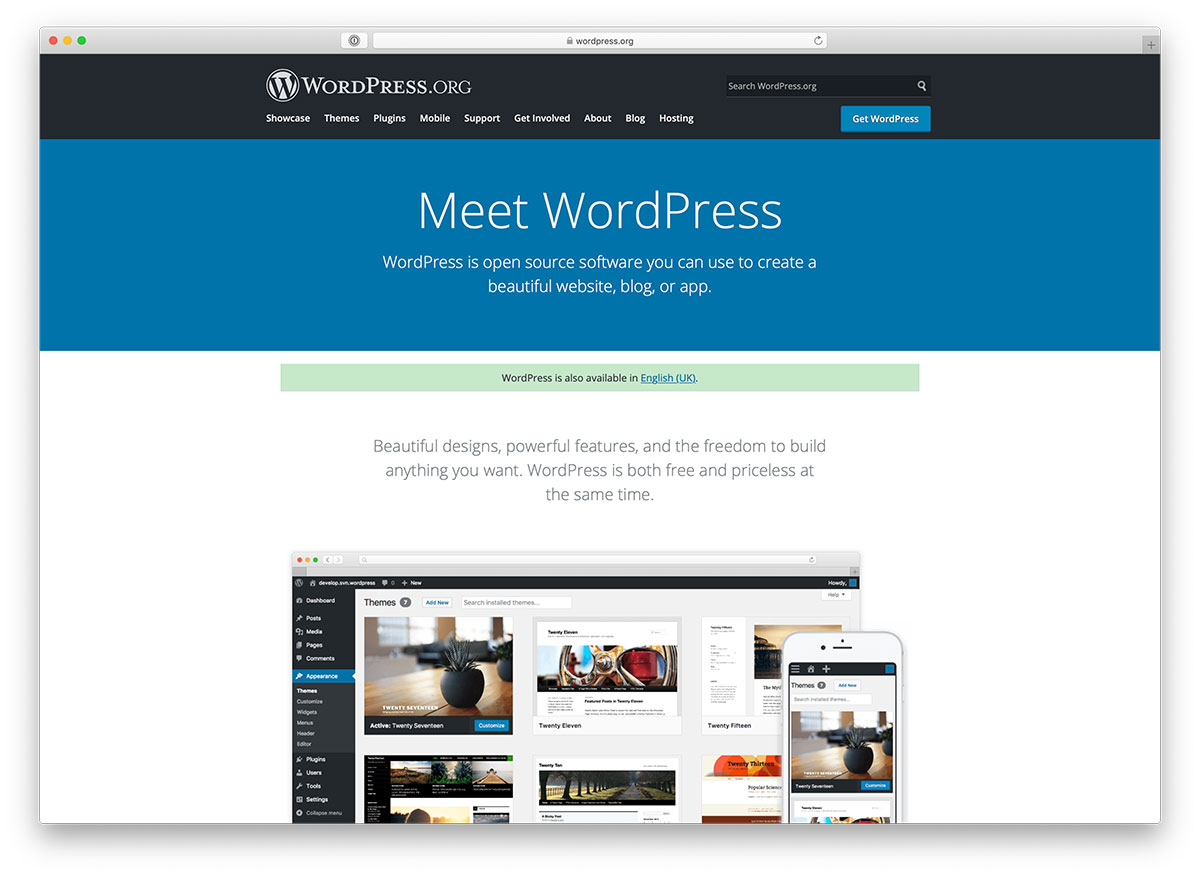The screenshot captures a detailed view of a browser window set to the WordPress.org website. 

At the top, the URL "wordpress.org" is visible in the browser's address bar, accompanied by the WordPress logo to the right of the bar. On the far left of the bar, three colored dots—red, yellow, and green—are present, signifying the browser's window controls.

To the right of the address bar, there is a small gray box with a dark gray plus sign inside. Directly below, a wide black header stretches across the page, featuring the WordPress.org logo toward the center-left. The horizontal navigation menu lists categories including: Showcase, Themes, Plugins, Mobile, Support, Get Involved, About, Blog, and Hosting. 

Towards the center-right of the header, there is a search bar labeled "Search wordpress.org" with a blue button labeled "Get WordPress" positioned just below it.

Beneath this header, the site unfolds into a prominent blue section with the text "Meet WordPress" centered within it. Following this, the phrase "WordPress is open source software you can use to create a beautiful website, blog, or app" is also centered.

The remainder of the page transitions into a white background featuring a large, centered gray rectangle at the top. This rectangle contains a hyperlinked text, "WordPress is also available in English (UK)". Below this, a statement reads, "Beautiful designs, powerful features, and the freedom to build anything you want. WordPress is both free and priceless at the same time."

At the end of the captured content, a visual depiction shows a browser and a smartphone displaying the WordPress interface.